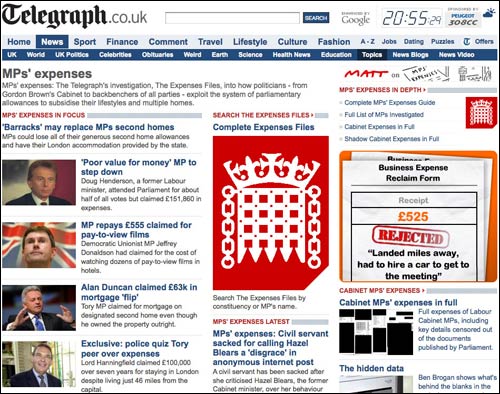This is an image of a webpage from The Telegraph (telegraph.co.uk). The logo "The Telegraph" is located in the upper left corner. To its right, there is an empty search bar with a blue search button labeled in white font; adjacent to the search bar is a note stating "Powered by Google." The timestamp "20:55" is displayed, and although some text on the right side is unreadable due to poor resolution, the main elements remain clear.

The site features a primary horizontal navigation menu with categories: Home, News, Sport, Finance, Comment, Travel, Lifestyle, Culture, Fashion, A-Z, Jobs, Dating, Puzzles, and Tea Offers. Below this is a secondary blue-colored navigation strip listing more specific sections: UK, World, UK Politics, Celebrities, Obituaries, Weird, Earth, Science, Health News, Education, Topics, News Blogs, and News Videos.

Prominently featured is an investigation titled "MPs' Expenses" by The Telegraph. The investigation delves into how politicians, from members of Gordon Brown's cabinet to backbenchers of all parties, exploit the system of parliamentary allowances to subsidize their lifestyles and multiple homes.